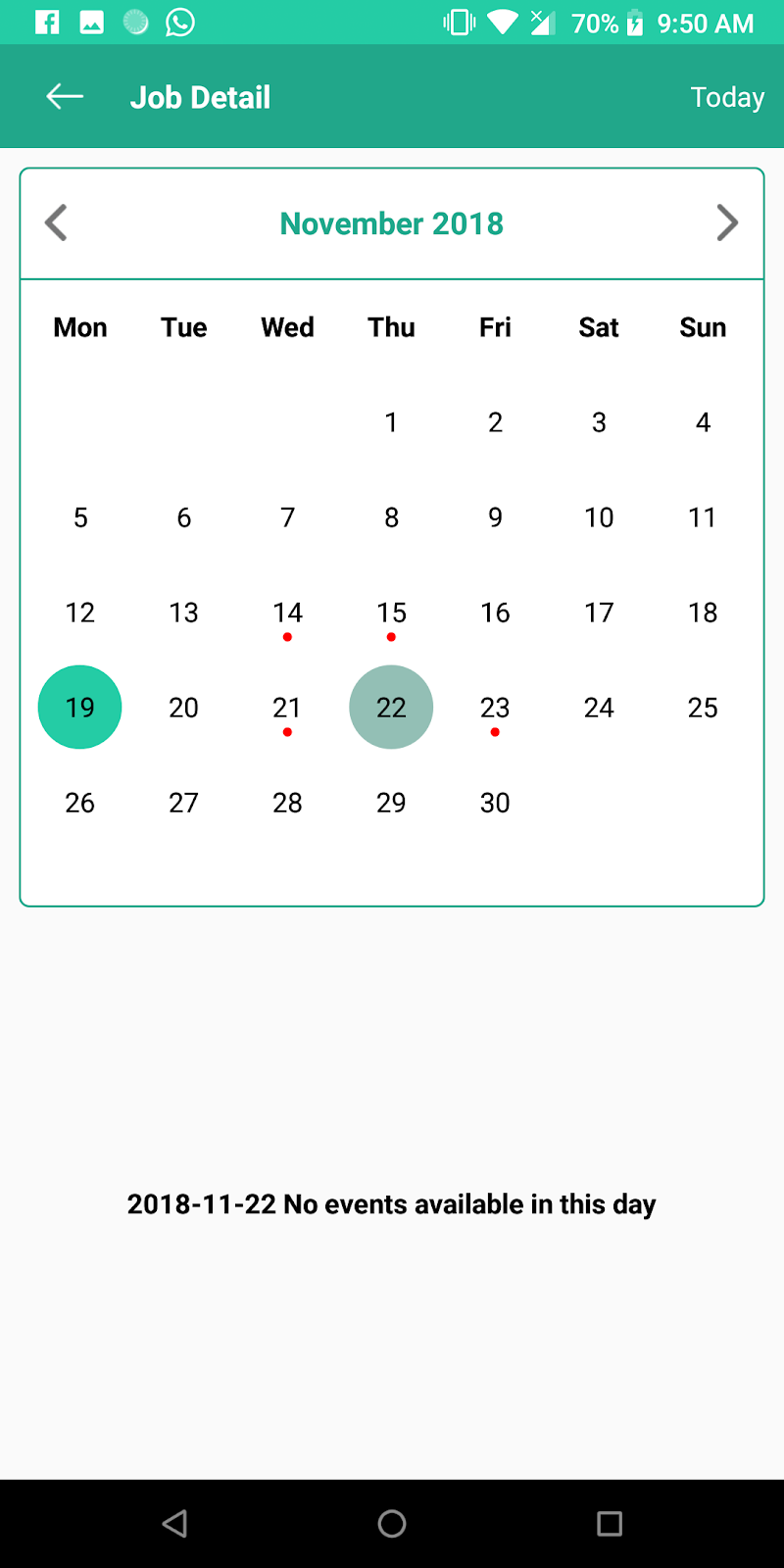The image showcases a smartphone screen with a detailed user interface. In the top left corner, icons for Facebook and phone options are visible. On the top right corner, status indicators for Wi-Fi, signal strength, and battery life (70% remaining) are shown, along with the clock displaying the time as 9:50 AM. The screen's background features a light green panel.

Below this, a larger, darker green panel is divided into two sections: the left side displays "Job Detail" in white text, while the right side shows "Today". Directly underneath is a calendar for November 2018, complete with arrows to navigate between months. The calendar, laid out from Monday to Sunday horizontally, spans 30 days.

Noteworthy details include the 19th and 22nd of November, which are encircled in green (with the 22nd in a lighter shade). Additionally, the 14th, 15th, 21st, and 23rd have small red dots beside their dates. Below the calendar, a message reads "2018-11-22. No events available on this day."

At the very bottom of the screen on a black panel, three navigation icons are present: a triangle, a circle, and a square.